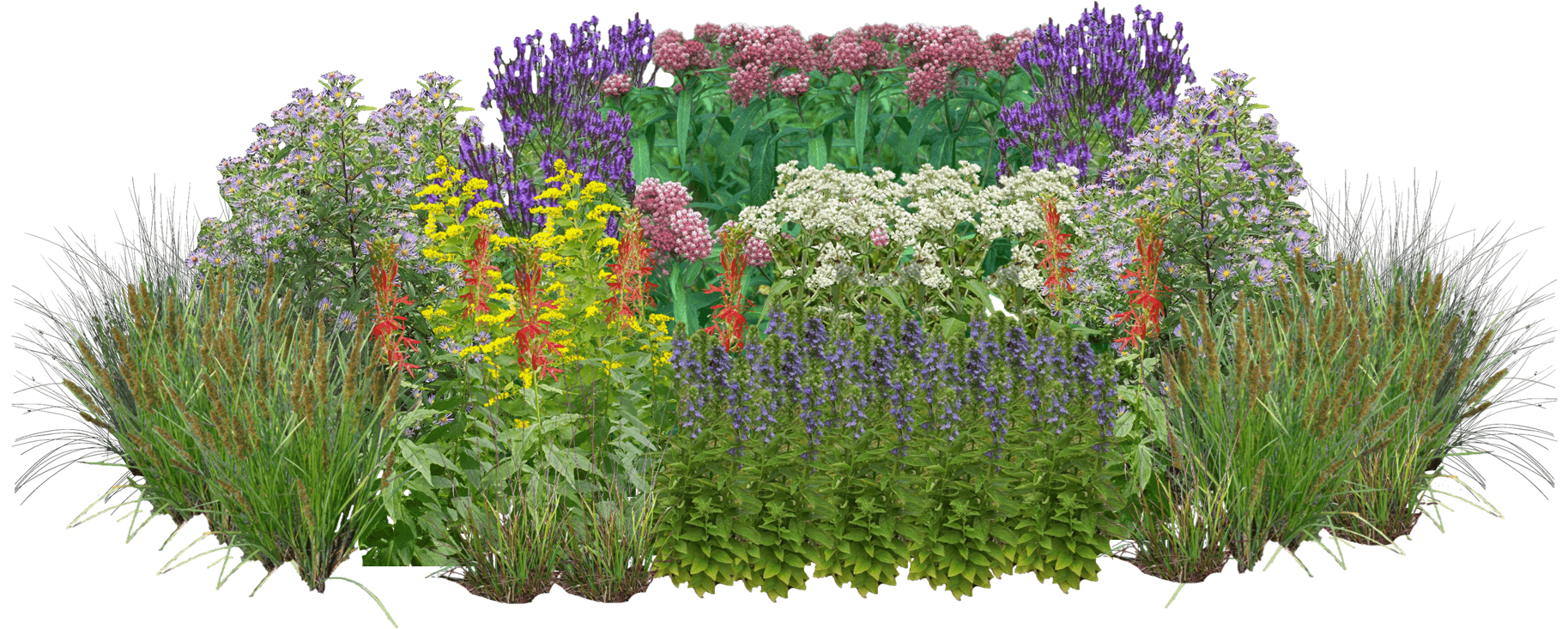This image showcases a beautifully arranged flower garden on a white background, featuring a variety of flowering plants and grasses in a symmetrical oval shape. The composition is layered, with the tallest plants at the back and shorter ones in the foreground, creating a visually pleasing gradient. Tall, spiky flowers with shades of purple and burgundy dominate the back row, potentially including species like lavender. In front of them, white blooms that resemble Shasta daisies are interspersed with other flowers, such as the light purple-pink alyssum. The middle section contains a mix of white, purple, and lavender flowers, while the foreground is adorned with vibrant red spiky flowers and some yellow and pink blossoms.

Ornamental grasses flank both sides of the garden, adding texture and framing the floral display. These grasses and the goldenrod, bee balm, and salvia plants scattered throughout enhance the garden's diverse and lush appearance. Overall, the arrangement is both aesthetically pleasing and richly colored with purples, pinks, whites, reds, and yellows, offering a harmonious blend of wildflowers and traditional garden flora.